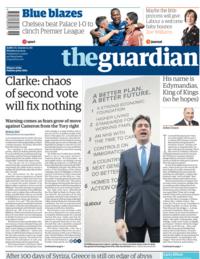The image depicts a page from a newspaper or magazine, predominantly white with black text. A blue bar approximately a quarter of the way down includes the title "The Guardian." At the top, several articles are visible, including one titled "Blue Blazes" in blue text, accompanied by an image of soccer players embracing. On the right, there is a picture of a woman, though the title above her is blurred.

Beneath "The Guardian" title, additional articles are listed. On the left, a headline reads, "Clark: Chaos of Second Vote Will Fix Nothing," followed by a subtitle and two columns of smaller text. In the middle of the page is a photo of a white man with dark hair, dressed in a dark suit and blue tie, appearing to speak with his mouth open. Behind him, a large text at the top reads "A Better Plan, A Better Future," and underneath are numbered points from one to six with corresponding text.

On the far right is an article about a man named "Edman," described as the "King of Kings," accompanied by a picture of this man in a suit, with additional text below.